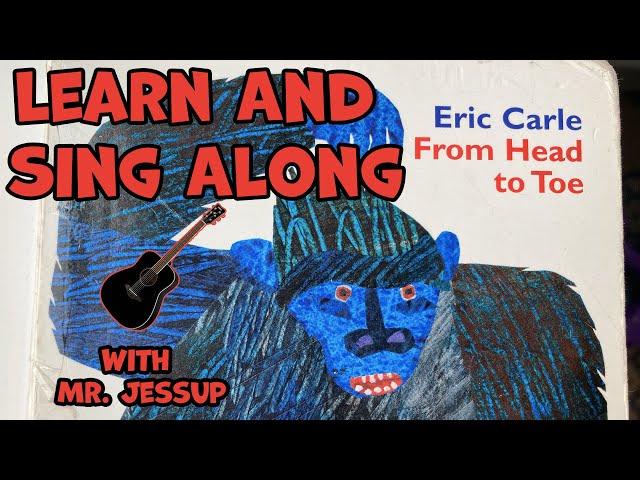The image is a cartoon-like illustration featuring a prominent, bold red text at the top left corner that reads "learn and sing along." The artist's name, Eric Carle, C-A-R-L-E, is inscribed in blue text on the upper right, accompanied by the phrase "from head to toe" in red text. At the bottom, in blue text, it says "with Mr. Jessup, J-E-S-S-U-P." The centerpiece of the drawing is a large, blue and black gorilla or sasquatch-like creature with a detailed, textured appearance. The creature has red eyes, a wide nose, an open mouth with visible white teeth, and one hand raised as if scratching its head. Additionally, there is a small graphic of a black guitar positioned near the creature's head, adding a musical element to the scene.